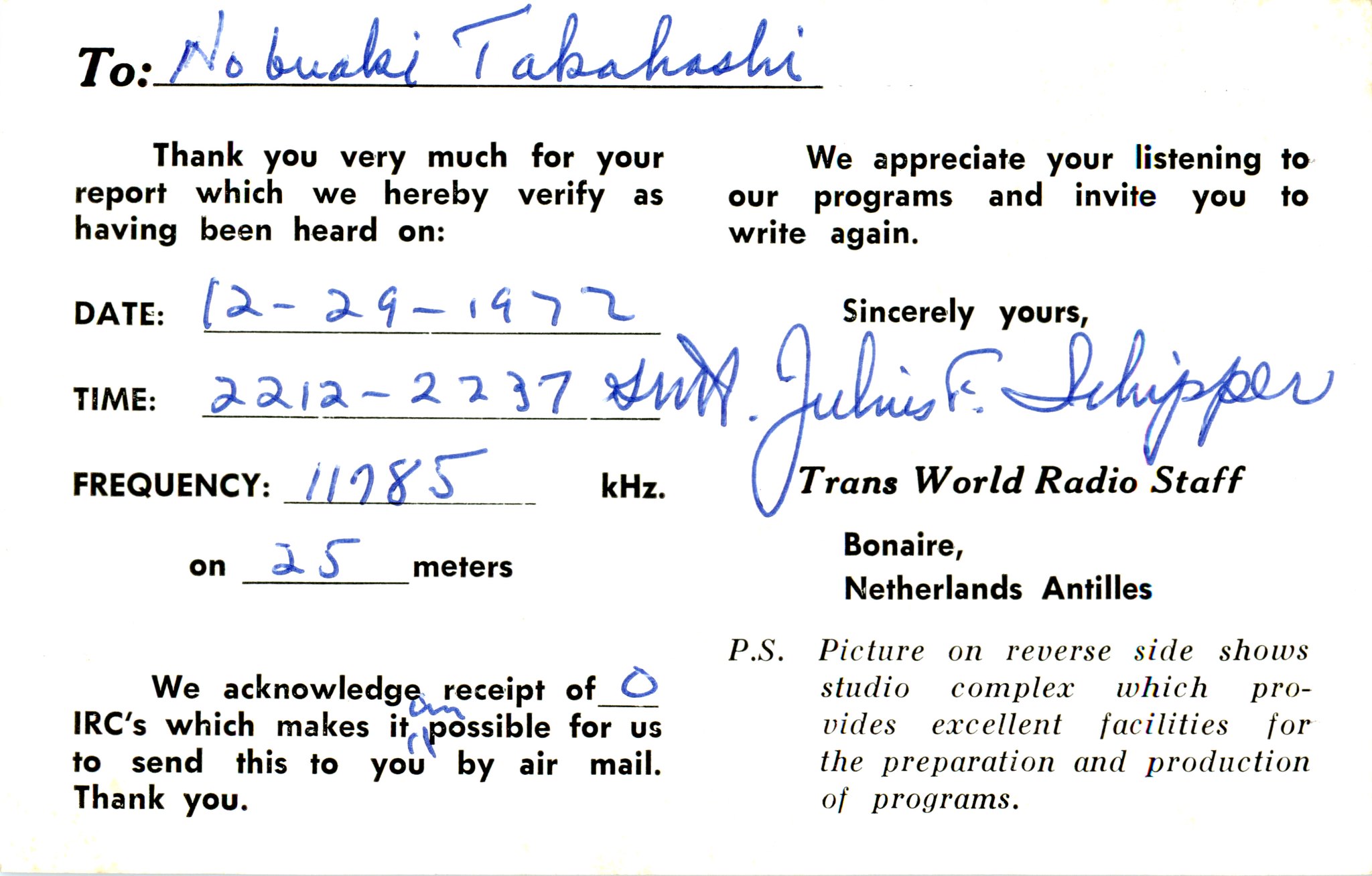The image depicts a letter addressed to Mr. Nobuki Takahashi from Trans World Radio staff member Julius F. Shippen, dated December 29, 1972. The letter thanks Mr. Takahashi for his report, which was verified with specific details: the report was heard at the time of 22:12-22:37 on the frequency of 11,785 kHz over 25 meters. The letter acknowledges receipt of zero International Reply Coupons (IRCs), making it possible to send the letter via air mail. The body of the letter is a mix of typed and handwritten text, with blue pen used to fill in certain fields. An additional note mentions that the picture on the reverse side shows the Studio Complex in Bon Air, Netherlands Antilles, which provides excellent facilities for program preparation and production. The letter ends by inviting Mr. Takahashi to continue listening and to write again, and is signed sincerely by Julius F. Shippen.